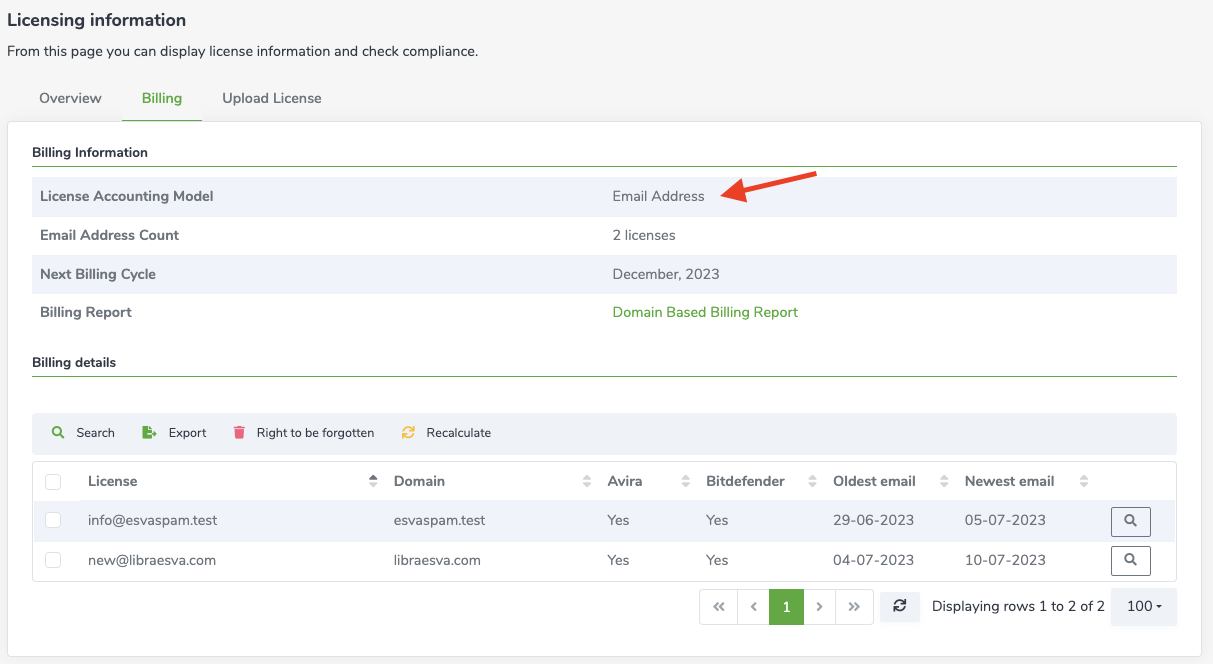The image depicts a webpage focused on licensing information, featuring various interactive elements and options. A prominent red arrow highlights the section where users are required to input their email addresses. The webpage includes functionalities such as 'Search,' 'Export,' 'Write to be Forgotten,' and 'Recalculate.' Additional sections displayed are titled 'Bilingual Welder,' 'Oldest Snail,' 'Newest Snail,' and names like 'Dominantasvaspim.test' and 'Librasfame.com,' suggesting associated platforms or categories. The billing report section outlines a 'Domain-Based Filing Report' with the next billing cycle noted as December 2023. Other specified fields include 'Email Address Count,' 'Incense,' 'License Accounting Model,' and 'Email Address.' The overall interface appears to be geared towards managing and reporting licensing and email-related data.